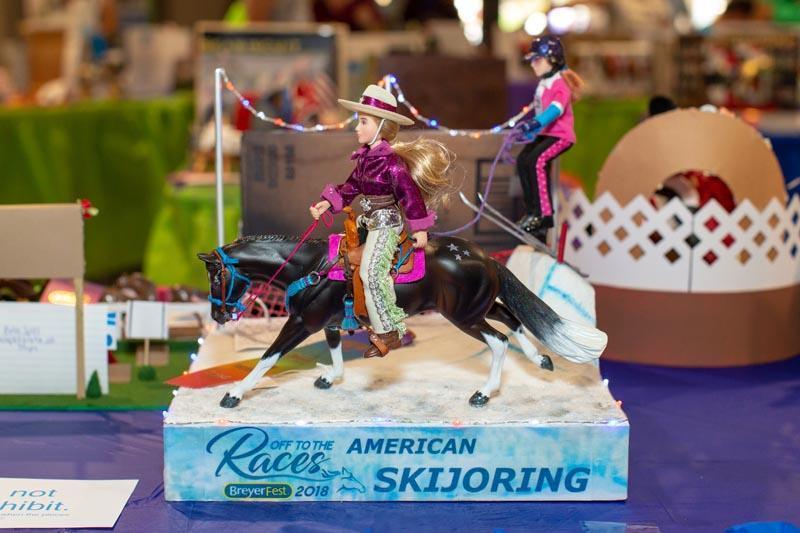This is a color photograph depicting a detailed miniature setup featuring two Barbie-like figurines engaged in a mock sport event called ski joring. The figurines are set on a turquoise platform with text that reads "Off to the Races, American Ski Joring" in blue font, and below it, in smaller print, "Briar Fest 2018." The centerpiece features a Barbie doll figurine riding a black toy horse with white legs and tail. This Barbie is dressed in a straw hat with a magenta ribbon, a purple shirt, and whitish pants. trailing behind her is another Barbie doll figurine on skis, connected to the horseback Barbie by a rope, suggesting she is being towed. The skiing Barbie is outfitted in pink attire, including a helmet. The entire setup is displayed on a table covered with a purple tablecloth. In the background, the blurred image reveals an ongoing event with other out-of-focus figurines and tables draped in green tablecloths, as well as some white lattice with brown framing. The scene is clearly staged for a specific celebration or display, emphasizing the intricate details of the Barbie figures and their constructed environment.